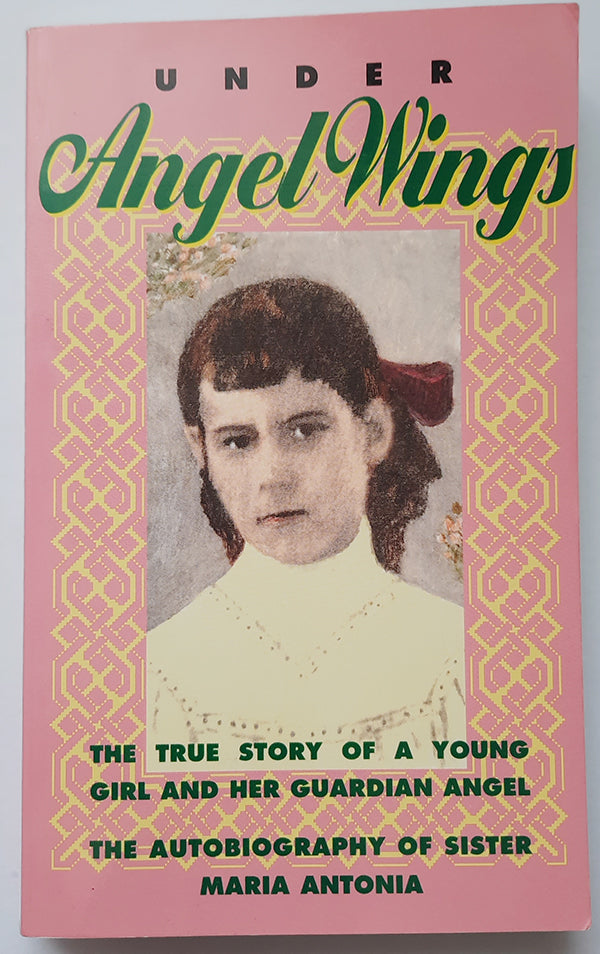The book cover is predominantly pink, featuring a central image of a young Caucasian girl with dark brown hair adorned with a red bow at the back. She has dark eyes and appears to be around eight or nine years old, wearing a high-neck white shirt paired with a red dress containing an indistinguishable pattern. The girl is looking slightly to the right. Above the image, in black text, is the title "Under" and below it, in fancy green text, is "Angel Wings." At the bottom of the picture, in green text, it reads, "The True Story of a Young Girl and Her Guardian Angel," followed by "The Autobiography of Sister Maria Antonia." Surrounding the image is an intricate geometric yellow frame, completing the aesthetically pleasing and detailed book cover.